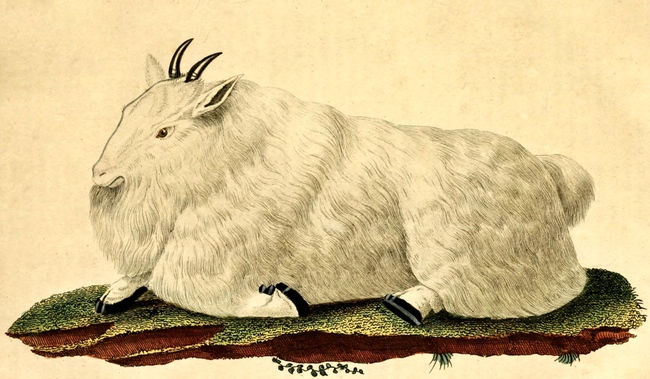The image depicts a large, white goat that looks somewhat like a cross between a sheep and a goat, lying down on a floating patch of green grass with a brown dirt underneath, which is interspersed with green leaves and blades of grass. The goat has thick white fur, black hooves, and prominent black horns on the top of its head. It strikes a relaxed pose, with one front paw extended forward and the other bent backward, a position echoed in its hind limbs. Its bushy tail and the goat's head turned to the side, gazing to the left, add to its serene demeanor. The background is a soft yellow or cream color, giving the image a smooth, parchment-like appearance, which somewhat isolates the goat and makes it the central focus. This detailed depiction creates an almost religious, iconic portrayal of the tranquil animal.